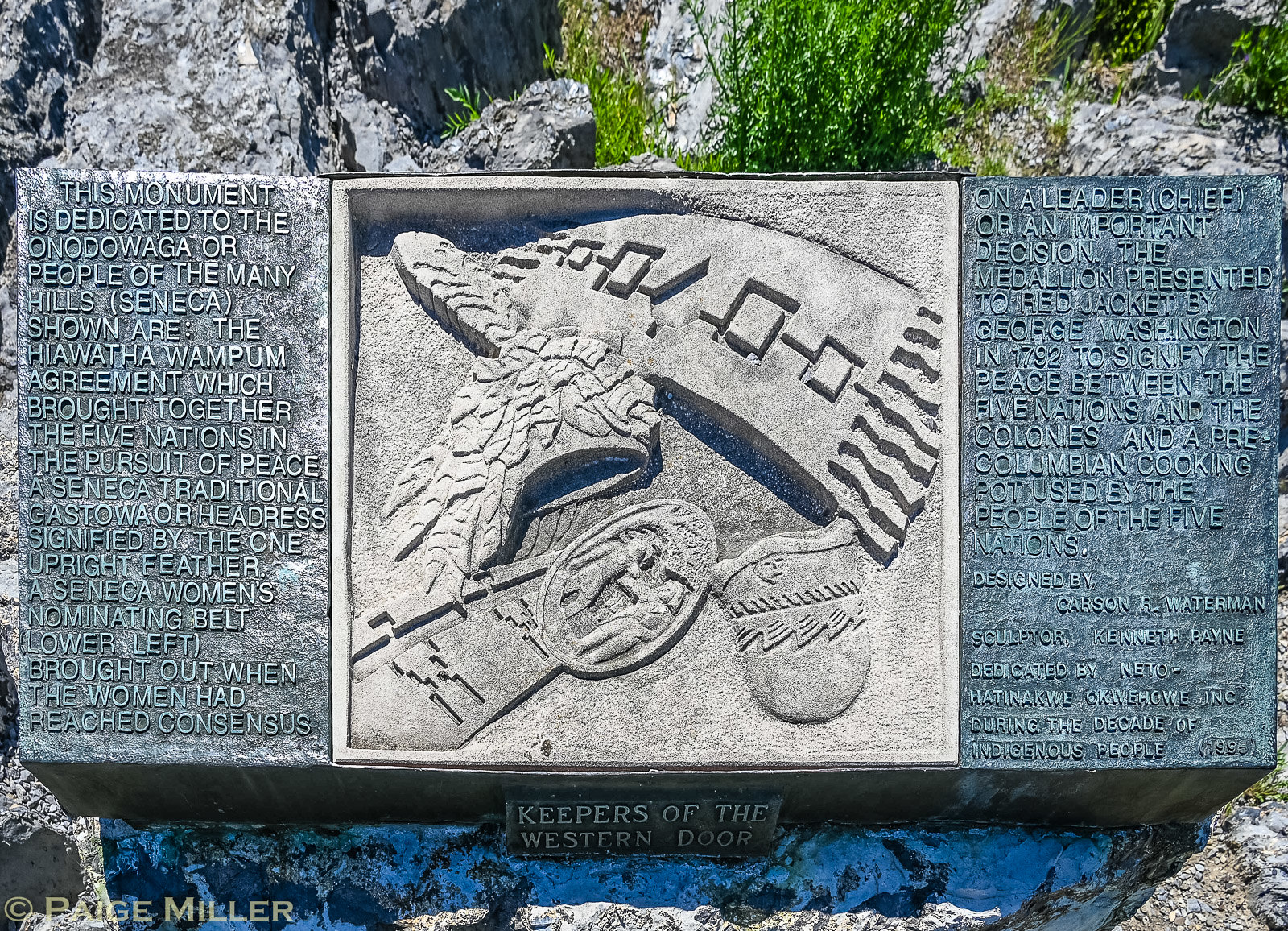This photograph captures a rectangular-shaped stone monument placed on a rocky and grassy ground, surrounded by green plants. The monument, crafted from a greenish stone, features intricate engravings and an embossed central illustration. The central part of the stone showcases a detailed image that includes elements such as an Indian head adorned with a traditional Kestoa headdress, distinguished by one upright feather. Surrounding this image are depictions of items resembling a pouch, belt buckle, and pendants, contributing to the intricately chiseled design.

On either side of the central image, capitalized English text is inscribed, detailing the purpose and significance of the monument. The left side of the text begins with a dedication to the Onöndowa’ga’ or People of the Great Hill (Seneca), noting the Hiawatha Wampum Agreement that united five nations in peace.

At the base of the monument, a small plaque reads, "Keepers of the Western Door." In the bottom left corner of the image, "Copyright Paige Miller" is visible, ensuring proper attribution to the photographer. The backdrop of the image is composed of more rock faces and greenery, enhancing the monument's serene and historical ambiance.